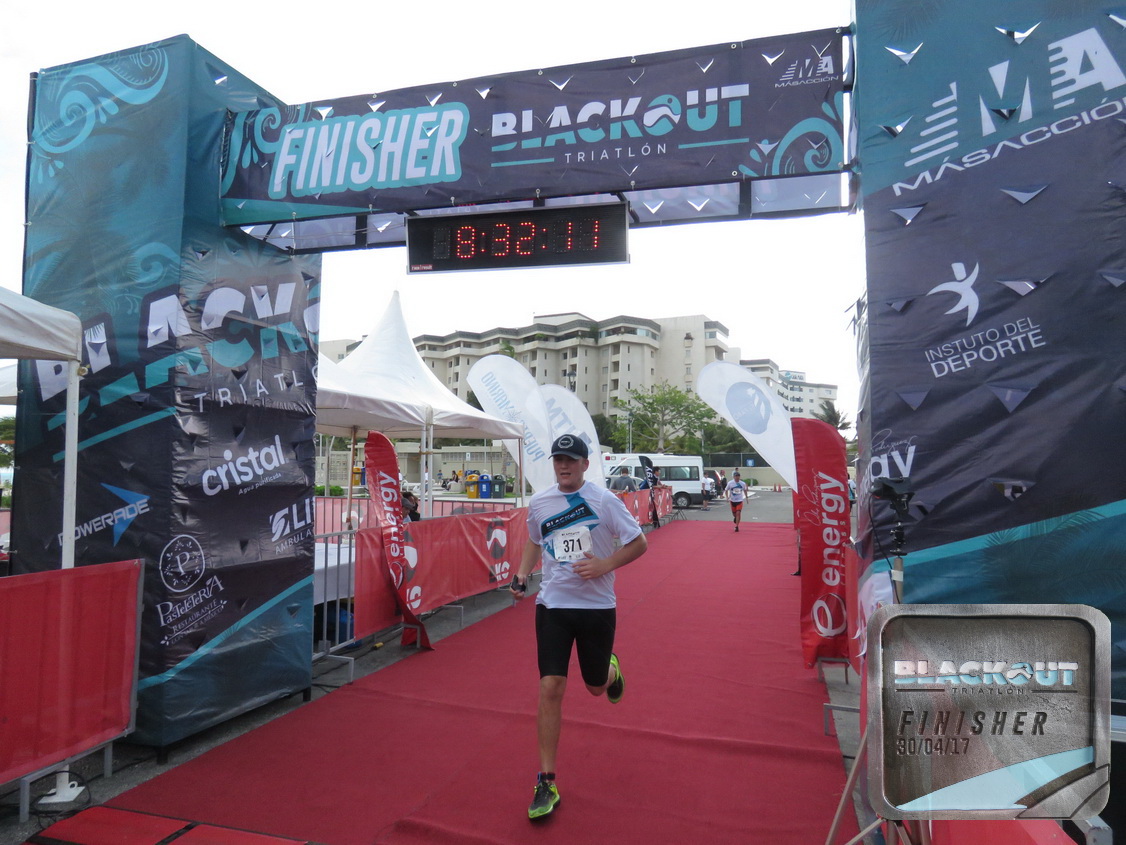The image captures a 45-year-old man running towards the finish line of the Blackout Triathlon. He is dressed in black shorts, a white top, and green shoes, with a black baseball cap and a white bib marked with the number 371. The runner is captured mid-stride on a red carpet-like mat under a large aqua green and black banner proclaiming "Finisher Blackout Triathlon." The timer above the runner shows 8 hours, 32 minutes, and 11 seconds. 

In the background, there is another man walking, along with visible emergency vehicles, vans, cars, and garbage cans, indicating a bustling finish area. Race officials are seen near white fences, with booths and a large building, possibly a hotel or apartment complex, further back in the scene. White and red flags line the sides of the marathon entrance, and it appears to be an overcast day.